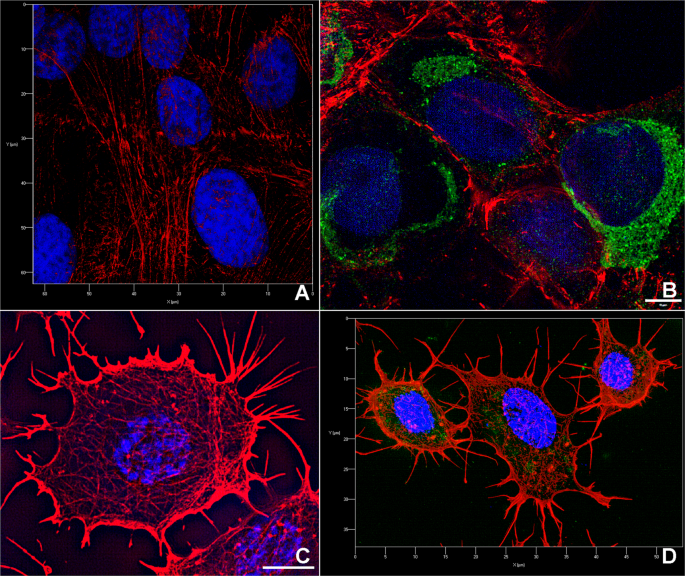The image is a composite of four microscope photographs, each depicting cells stained with vibrant colors to highlight different features. The top left panel (labeled A) shows a grid overlay with numerical scales ranging from 0 to 55 on the bottom and 0 to 80 on the left. This section displays a network of delicate red veins interspersed with large blue ovals. The top right panel (labeled B) reveals similar red veins with blue ovals, but these are further surrounded by green areas, making this section more colorful and complex. The bottom left panel (labeled C) captures an amorphous red blob with a distinct blue circle at its center, showing a closer and more detailed view. The bottom right panel (labeled D) seems to be a wider, less detailed shot similar to C, showing the same type of cells but from a different angle or distance. The blue markings in panels C and D are particularly striking, resembling glowing thumbprints. Despite the colorful differences, all panels appear to originate from the same cell culture, providing varying perspectives and magnifications of the cellular structures.